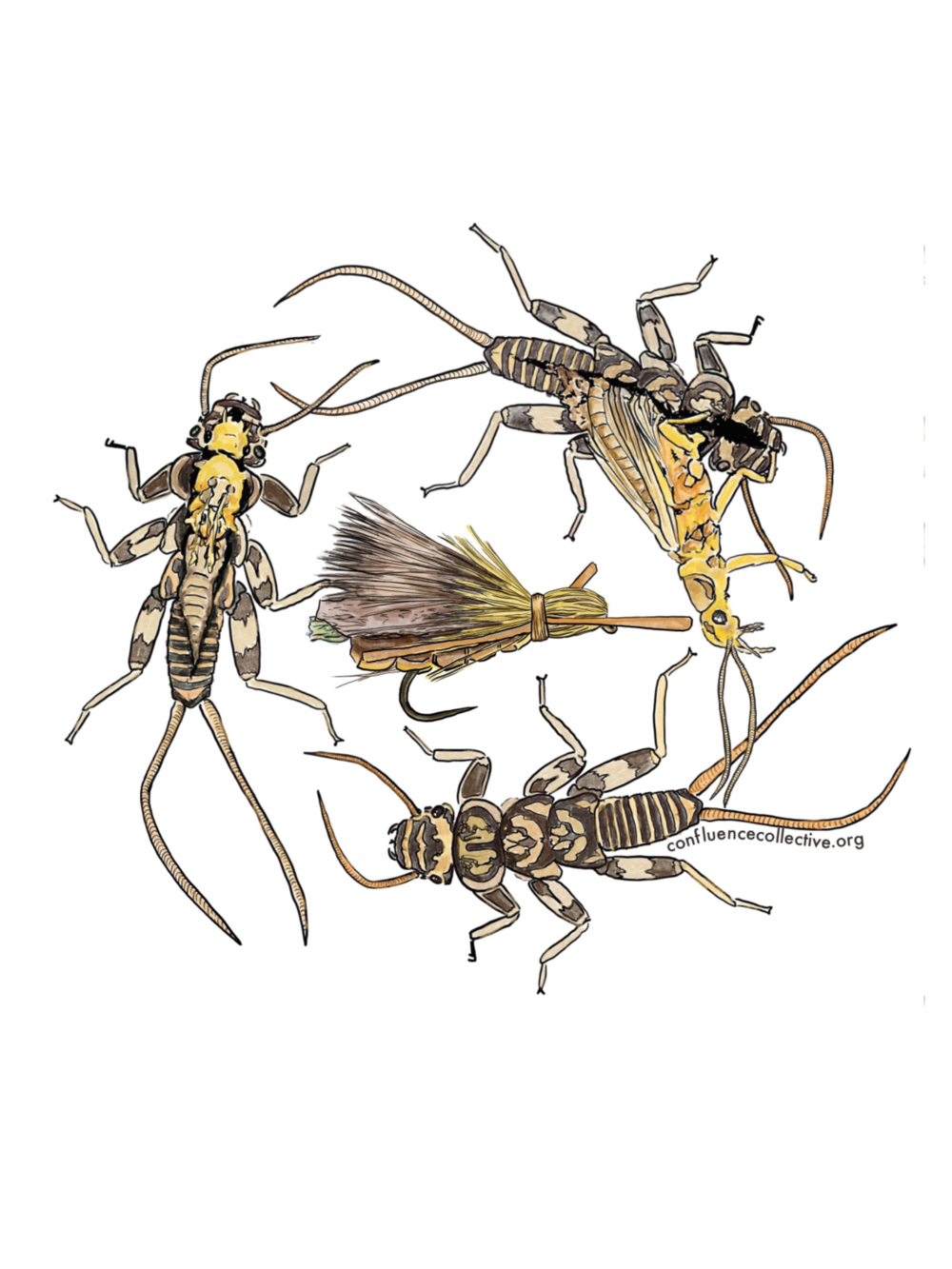The illustration features detailed and colored drawings of various insects, most closely resembling locusts or grasshoppers, all depicted with six legs and antennas. These insects are primarily colored in shades of brown, black, yellow, and even some light green. The insects are intricately arranged in a circular pattern on a white background, leading to a central focal point that appears to be a handmade fishing fly, complete with feathering and a large, curved hook. This fly, likely intended to catch fish, adds a dynamic element to the composition. One of the insects is shown in various stages of molting, breaking through its exoskeleton. At the very bottom of the illustration, beneath one of the bugs, is the URL "confluencecollective.org," suggesting the source or artist of the work.